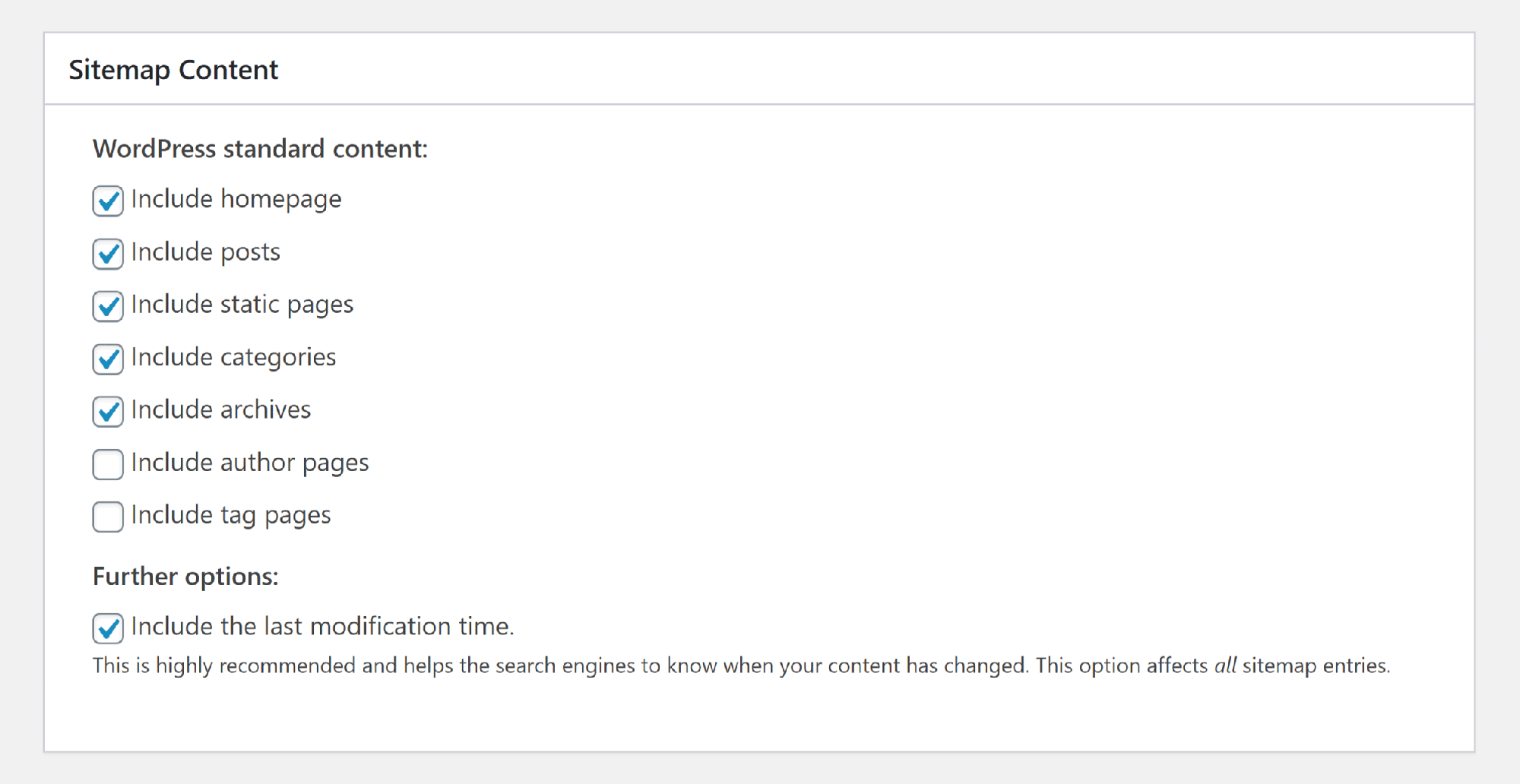The image showcases a settings interface for configuring a sitemap in a WordPress environment, presented against a neutral gray background. The interface primarily appears in shades of green, blue, and gray, and it includes various options related to the sitemap content.

1. **Checkboxes for Sitemap Content:**
   - **Homepage**: The option to include the homepage is selected, indicated by a blue check mark.
   - **Posts**: This checkbox is also checked, meaning posts will be included in the sitemap, as denoted by the blue check mark.
   - **Static Pages**: Marked by a blue check, static pages are set to be included.
   - **Categories**: This option is checked, ensuring categories are part of the sitemap.
   - **Archives**: With a blue check, archives are included in the sitemap.
   - **Author Pages**: An option to include author pages exists but is currently unchecked.
   - **Tag Pages**: The checkbox for tag pages is available but not selected.

2. **Further Options Section:**
   - **Include the Last Modification Time**: A crucial setting, indicated by a blue check mark, recommends that the last modification time is included for each entry in the sitemap. This feature helps search engines better understand when content has been updated. It affects all sitemap entries, as emphasized in italics.

Additional context notes that the setting of including the last modification time is highly recommended to aid in search engine optimization, highlighting its importance in keeping search engines informed about the latest updates to the website's content.